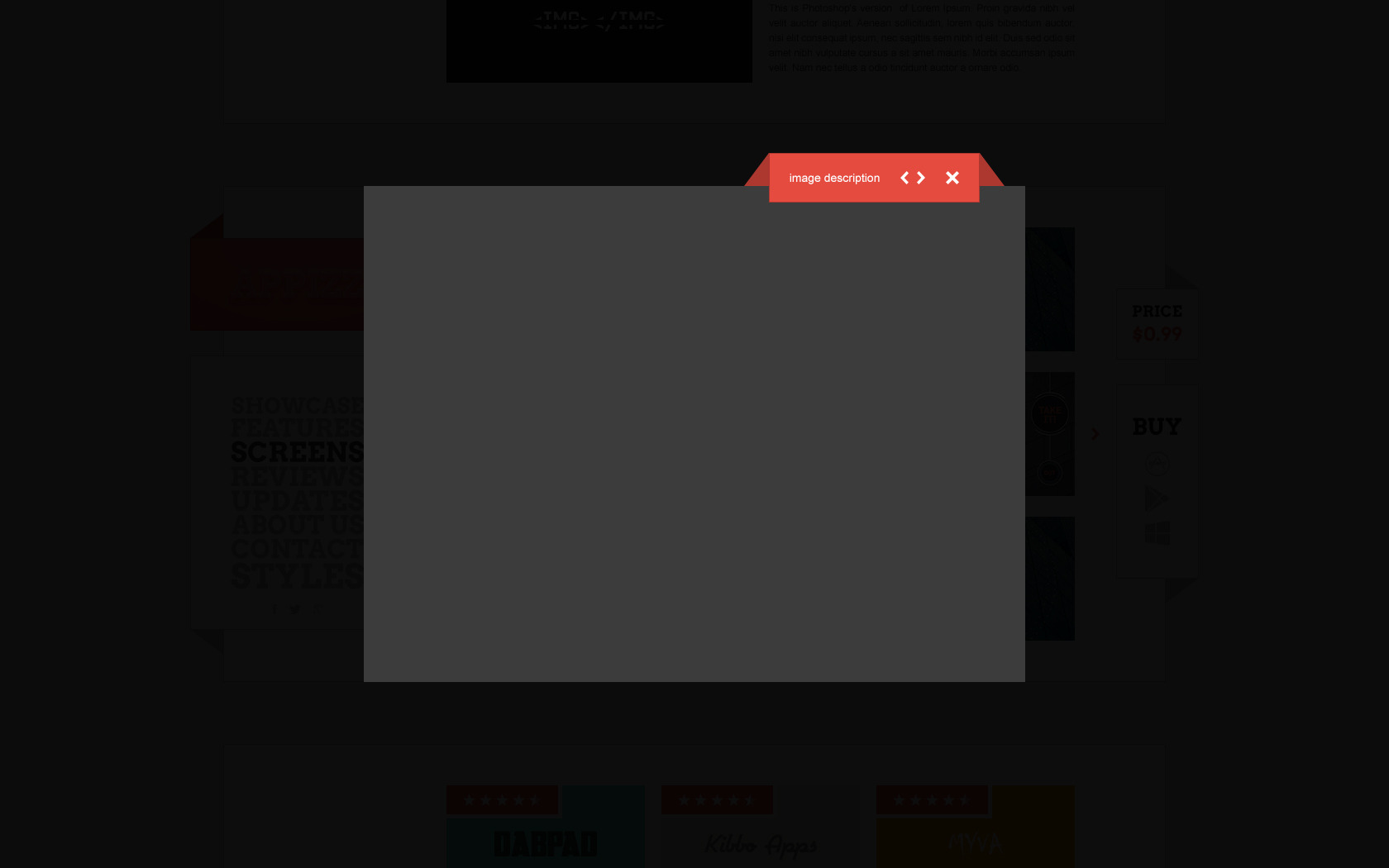The image depicts a minimalist digital interface. Dominating the scene is a large, solid black rectangle that serves as the background. Centered within this black expanse is a smaller, light gray rectangular pop-up. In the top right corner of this gray rectangle, there is an icon featuring a folded design resembling a piece of paper, which appears to float slightly above the right-hand side but not touching the edge.

Within the pop-up, the text "Image Description" is prominently displayed in white. Directly to the right of this text are three distinctive icons: a white back arrow, a white forward arrow, and a white X, presumably for navigation and closing the pop-up. The overall design is stark and devoid of additional elements such as search bars, login fields, or web addresses, maintaining a clean and uncluttered visual focus.